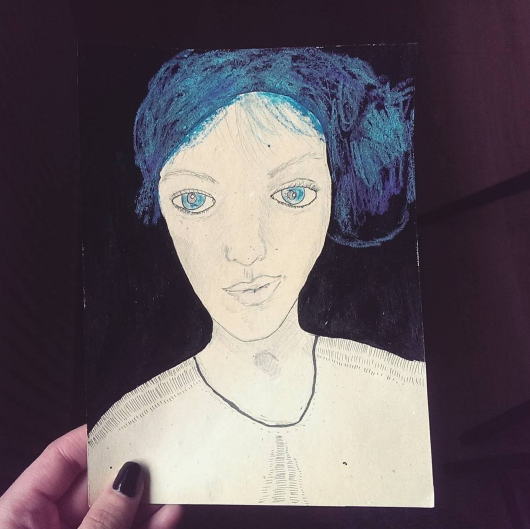The image depicts a digital photograph of a hand-drawn portrait being held by a Caucasian person. The hand in the lower left corner has a dark red painted thumbnail. The background in both the photo and the drawing is almost pitch black. The portrait itself is of a white woman with an oval-shaped face, large, oval blue eyes, and blue-purplish hair that is tied up and parted more to the right. The woman has a fairly large nose, a smirk-like smile, and thin eyebrows. The artwork is rendered in shades of gray pencil and crayon, with some areas appearing unfinished. She is wearing a thin necklace and a V-neck shirt with detailed lines on the shoulders.